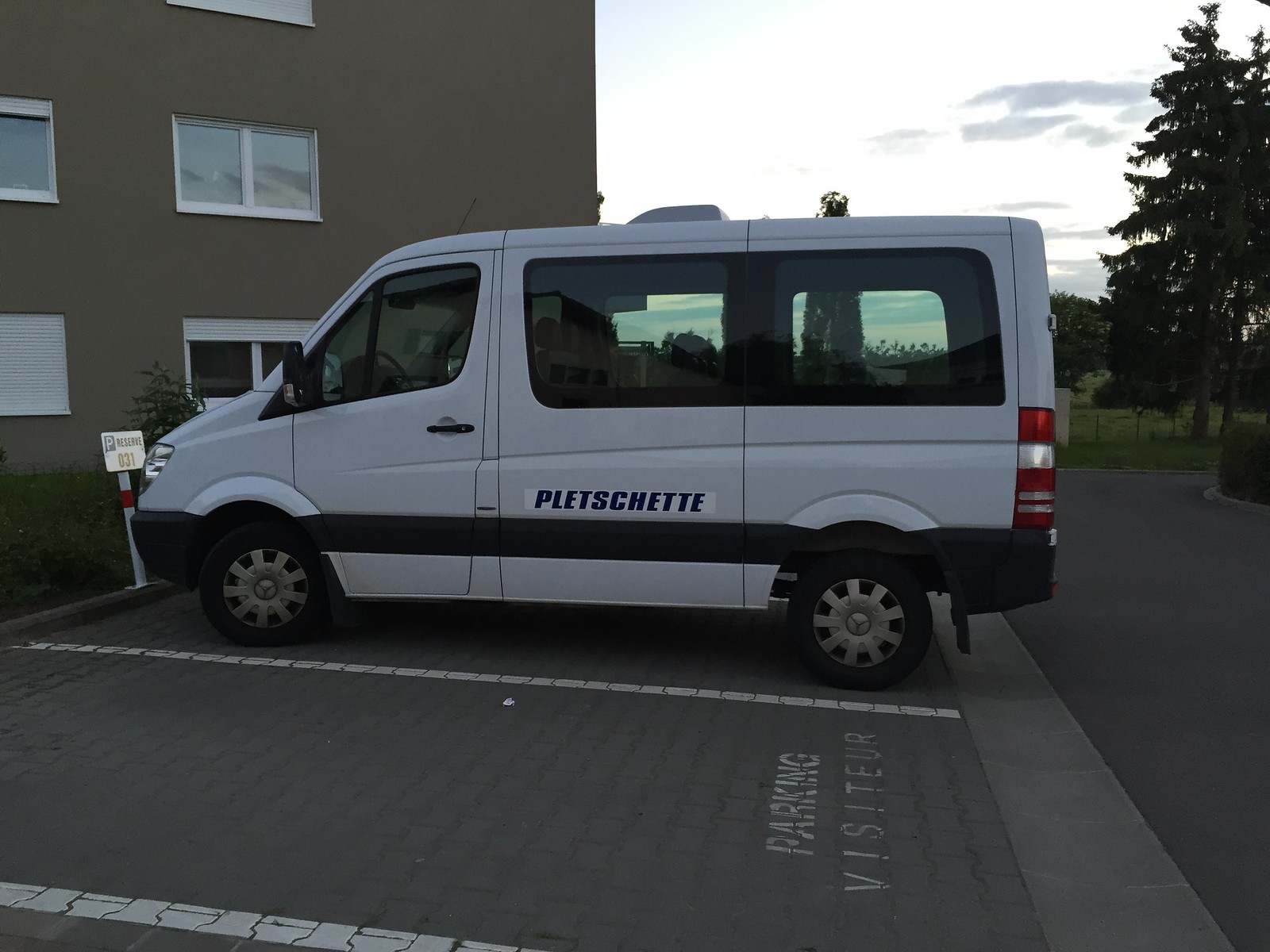In this side view photograph of a late-afternoon outdoor setting, we see a white van with a black stripe along the bottom, parked in one of two visible parking bays made of brick pavement. The text "Parking Visitor" is stenciled in white within the bay holding the van. The adjacent bay is empty. The van faces left and is stationed in front of a multi-storied, rectangular gray building with multi-paned, white-framed windows. A sign near the parked van displays a "P" and suggests a reserved spot, though finer text detail, including "reserve 031," is not fully legible in the image. In the distance on the right side, a green pine tree stands tall against a sky that is light blue and white with dark gray clouds, indicating that it is nearing dusk.